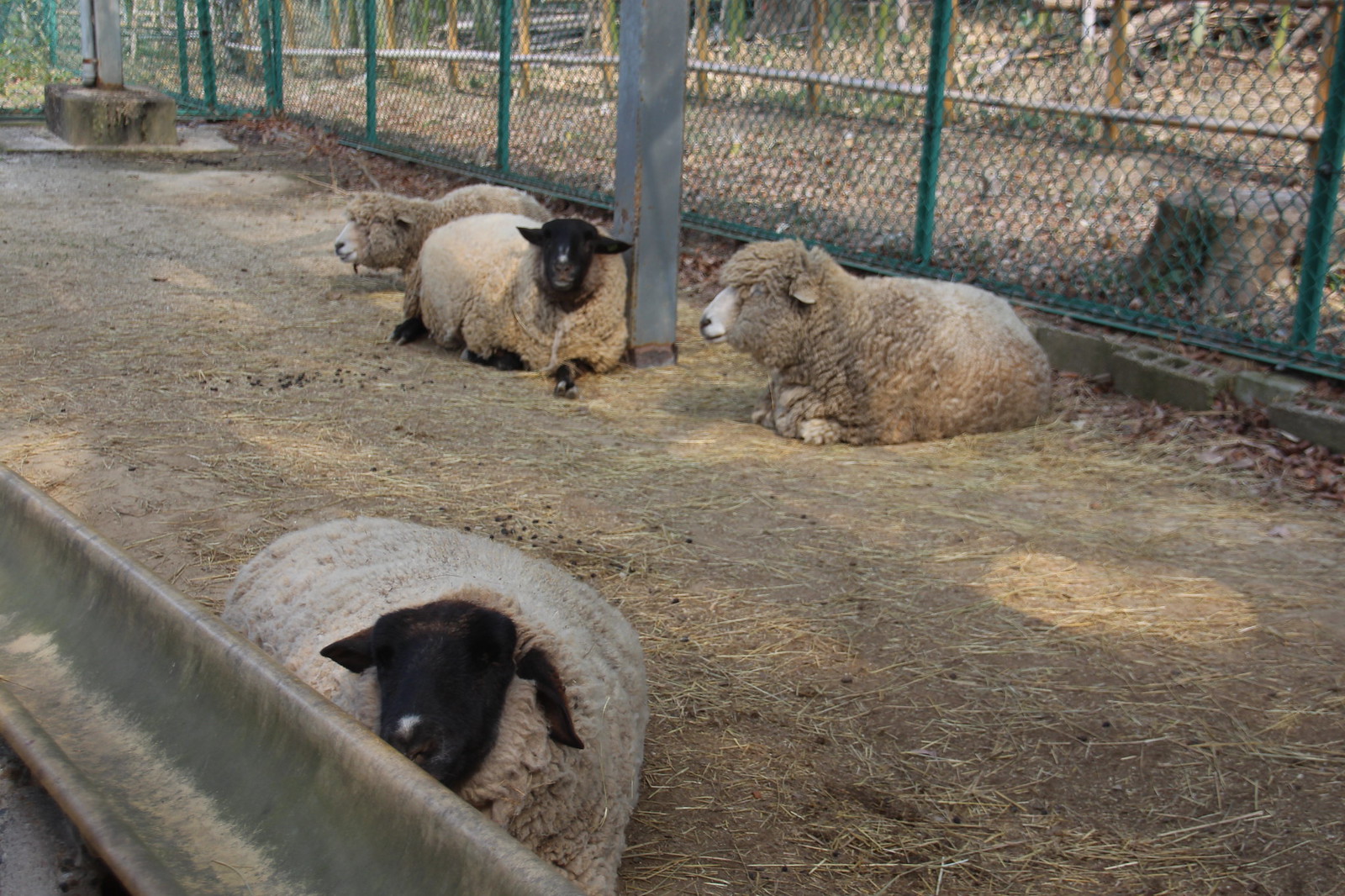This slightly blurry digital photograph depicts an outdoor sheep paddock with four unshorn, woolly sheep lounging on a dirt ground sparsely covered with straw. Of the four sheep, two have black faces and two have white faces, with one particularly close to the camera, peering directly at the lens. In the foreground, there's a metal feeding trough positioned on the lower left side, possibly containing remnants of sheep feed. The enclosure is secured with a green chain-link fence, and further behind is a brown wooden fence punctuated by upright wooden pillars. The ground within the paddock is a mix of dirt, straw, and scattered debris. A gray metal pole stands almost centrally in the background, and in the upper left corner, a bale of hay is partly visible. The overall scene suggests a neglected, somewhat untidy environment, emphasizing the need for the sheep to be shorn.